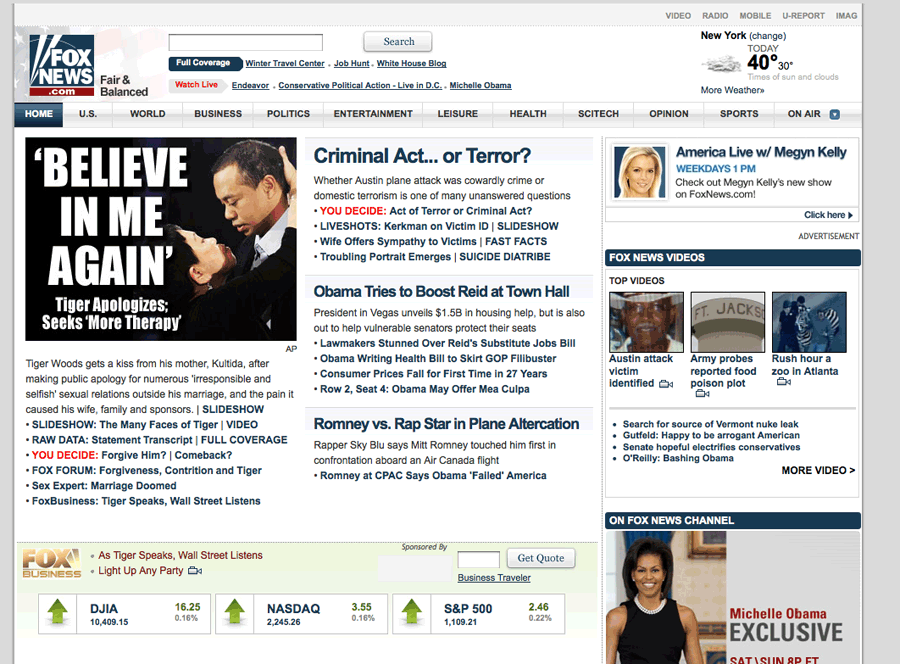The Fox News website homepage features a predominantly white and blue color scheme with the slogan "Fair and Balanced" prominently displayed. The top navigation bar includes a search function, current weather conditions for New York, and a link to a detailed weather report. Additional links in the menu guide users to sections like the Winter Travel Centre, Job Hunt, and the White House Blog, among others.

The main story on the page is centered around Tiger Woods, with the headline reading "Believe in Me Again as Tiger Apologises and Seeks More Therapy." The accompanying article details that Tiger Woods received a kiss from his mother after issuing a public apology for his numerous irresponsible and selfish sexual relationships outside his marriage, acknowledging the pain caused to his wife, family, and sponsors.

Other notable stories include a piece titled "Obama Tries to Boost Read at Town Hall," and an exclusive feature with Michelle Obama located in the bottom right corner. The top right corner of the page advertises "America Live with Megyn Kelly," airing weekdays at 1 p.m.